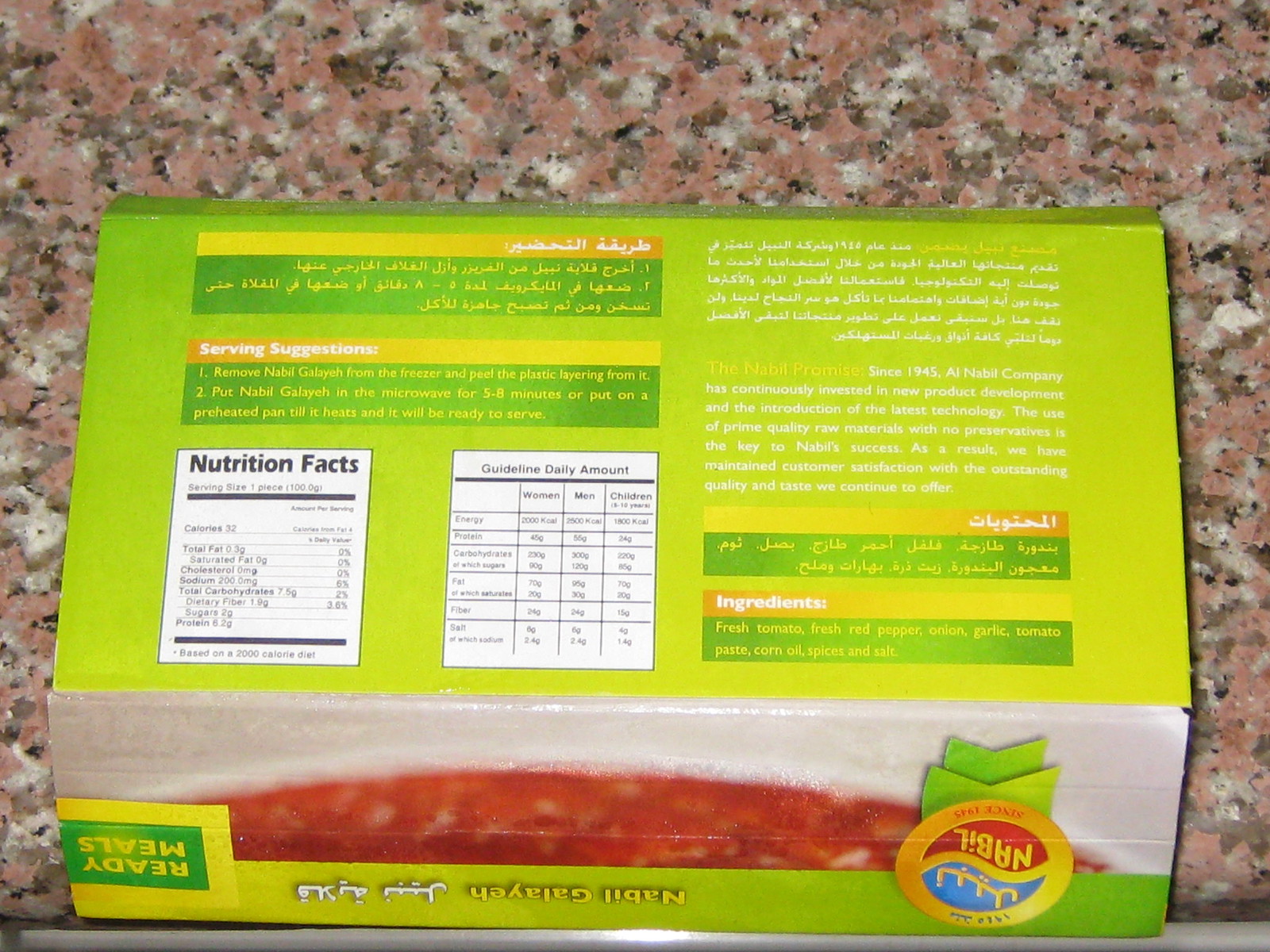The image depicts a green box of food, specifically a Ready Meals package from the company Nabil, placed on a marble countertop with pinkish and whitish tones. The box displays both Arabic and English text, prominently showing serving suggestions and nutritional information. The serving suggestions instruct to either microwave the meal for five to eight minutes or heat it in a preheated pan. The meal appears to be a tomato-based soup, with ingredients listed as fresh tomatoes, fresh red pepper, onion, garlic, tomato paste, corn oil, spices, and salt. The box, photographed from an angle, has light gleaming off it, causing some blurriness. On the side of the box, there's an image depicting the prepared soup.